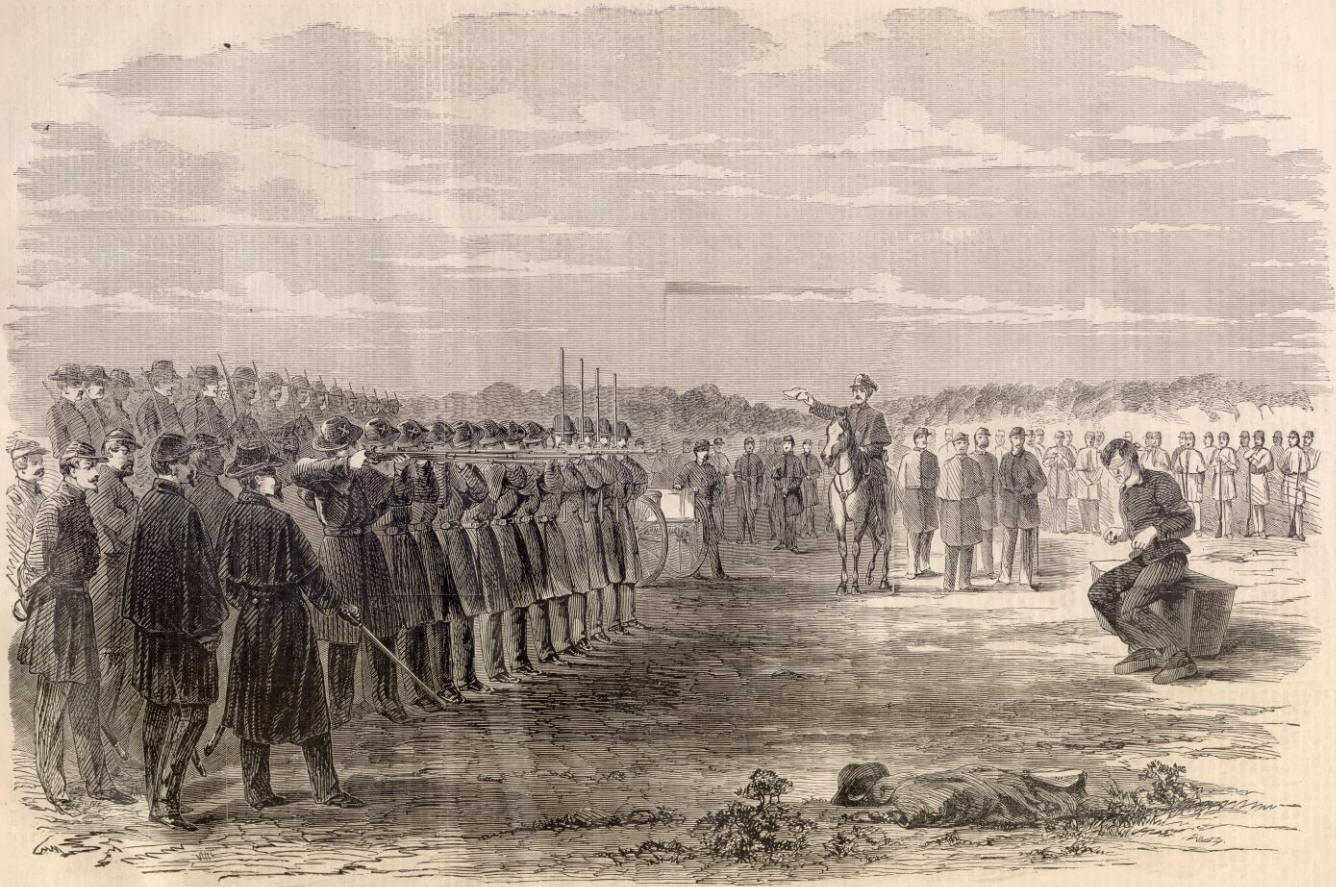The image is an intricate black-and-white drawing resembling a vintage pen and ink illustration, likely a print from an old magazine or newspaper. The scene depicts a historic military event, possibly an execution by a firing squad. The upper half of the image is dominated by a cloudy sky rendered with a delicate grid of dots, giving it a woven appearance.

At the center of the drawing sits a man dressed in dark clothing, seemingly bound in chains, perched on a large stone or block. His posture is dejected, with bent knees and bowed head. Surrounding him in the foreground are possible remnants of fallen bodies, identifiable by bits of cloth and skeletal outlines, amidst some patches of dirt and weeds.

To the left side of the image stands a line of soldiers in dark, period-appropriate uniforms, reminiscent of the Civil War or Revolutionary War era. They hold old-fashioned rifles, some aimed directly at the seated man while others are raised vertically. The soldiers' uniforms consist of belted coats extending just below the knees, dark pants, and hats, and many sport mustaches and beards.

In the mid-ground, a man on a white horse commands attention. He wears dark clothing and possibly a ranger hat, holding up what looks like a white handkerchief or flag, as if signaling an order. His angled position and authoritative gesture suggest he is directing the soldiers.

Further back, faint lines of additional men and a probable cannon can be observed, adding depth to the scene. This rear group appears more faded, enhancing the sense of distance and scale. The horizon is punctuated with the outline of a mountain range, also rendered in gray, completing the grim, tense atmosphere of this historic battlefield tableau.